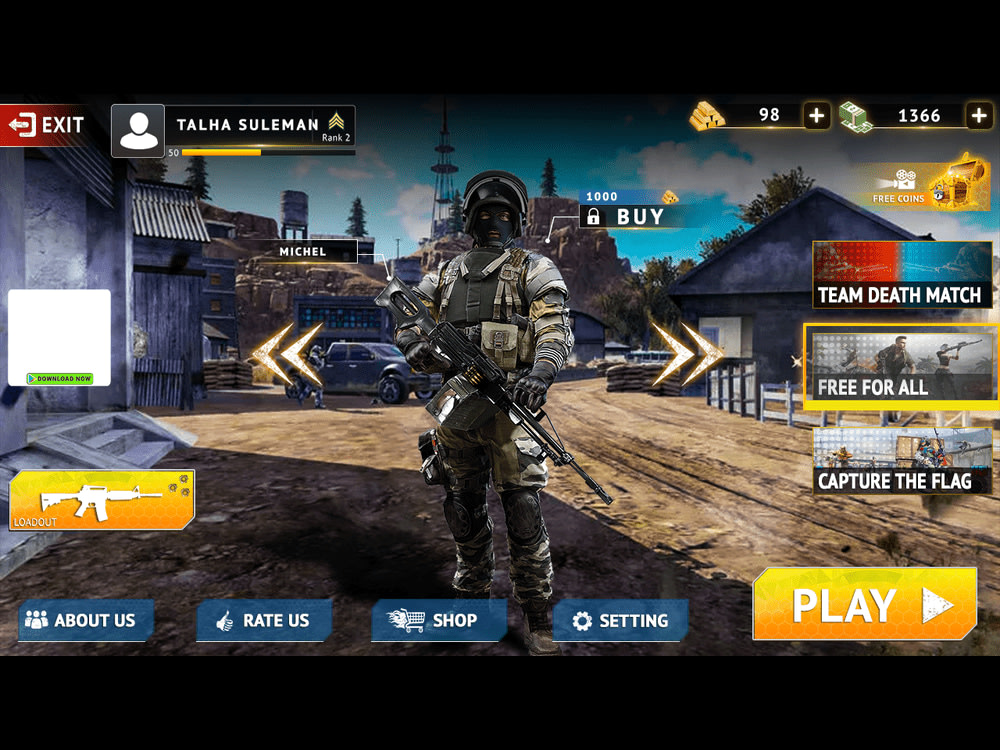This image is a detailed screenshot from a combat-themed video game. Central to the frame is a soldier, the playable character, dressed in full camouflage combat gear, including a bulletproof vest, helmet, and ski mask. The soldier is also equipped with various accessories, packs, and weaponry, prominently holding an automatic rifle. Extra gear, possibly including bombs or additional firearms, is strapped to his side. 

The screen displays various in-game statistics and options. On the top left, there's a red "Exit" button next to the player's name, "Talha Suleman," spelled out as T-A-L-H-A S-U-L-E-M-A-N. Moving right, the interface shows in-game currency represented by gold bars labeled '98' and stacks of money totaling '1,366'. Below these, the game modes "Team Deathmatch," "Free-for-All," and "Capture the Flag" are listed.

At the bottom of the screen, there are four blue rectangular buttons marked "About Us," "Rate Us," "Shop," and "Settings." On the far right, there's a prominent orange-yellow triangular "PLAY" button. The background depicts a war-torn environment with concrete buildings, vehicles like F-150 trucks, and sparse vegetation, suggesting an abandoned town overtaken by conflict. There are no other characters visible, emphasizing the lone soldier poised for action.